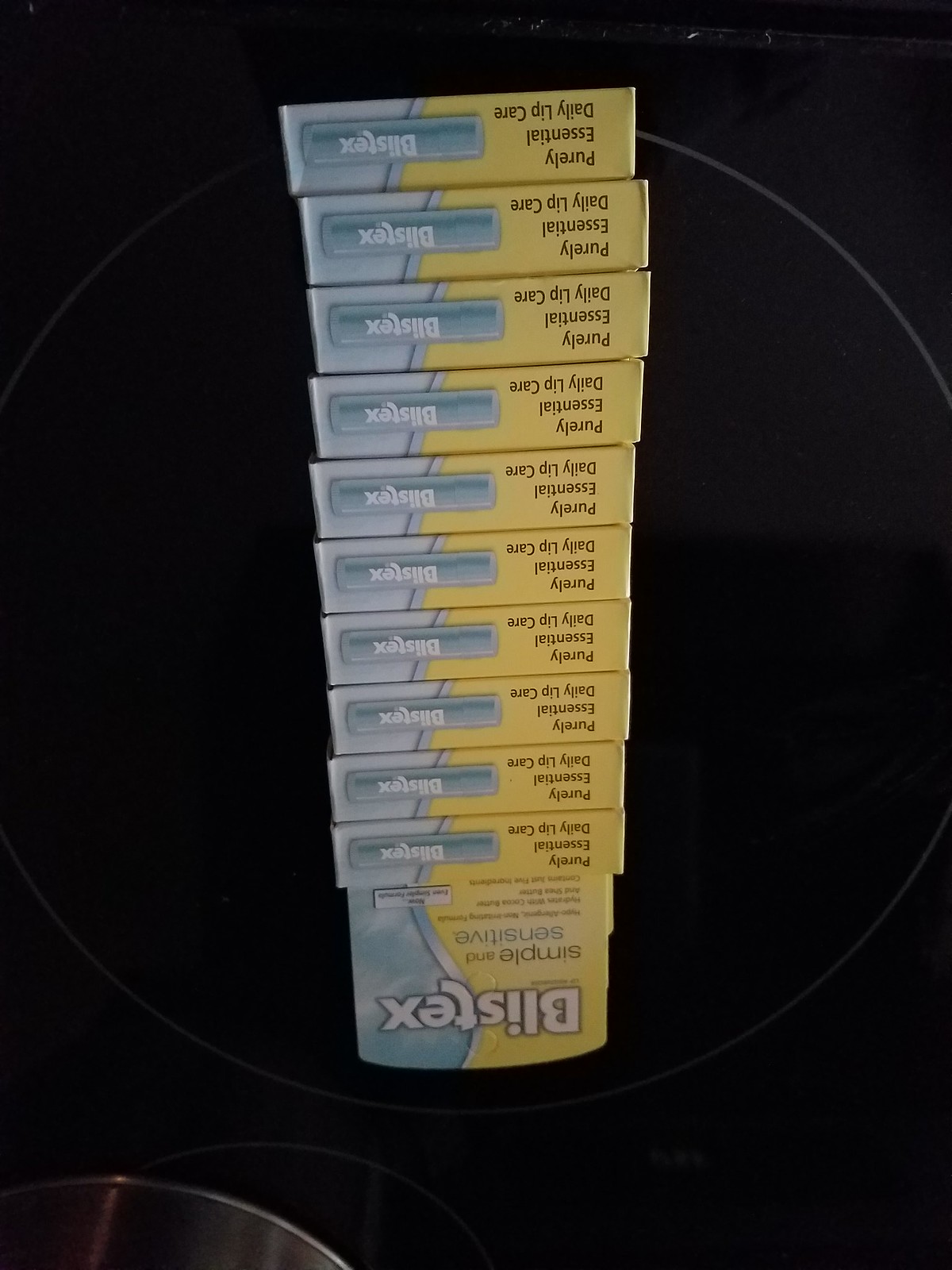The vertical rectangular photograph features a black background resembling a stove top with gray circular outlines suggestive of burners. Centrally stacked are approximately 10 to 12 upside-down Blistex packages. Each package is half yellow and half aqua blue-green, with white text reading "Blistex" along with black writing. Prominently displayed on the boxes are phrases like "Simple and Sensitive" and "Purely Essential Daily Lip Care." The Blistex containers themselves echo the blue-green hue and white writing of the packaging, creating a cohesive product display.